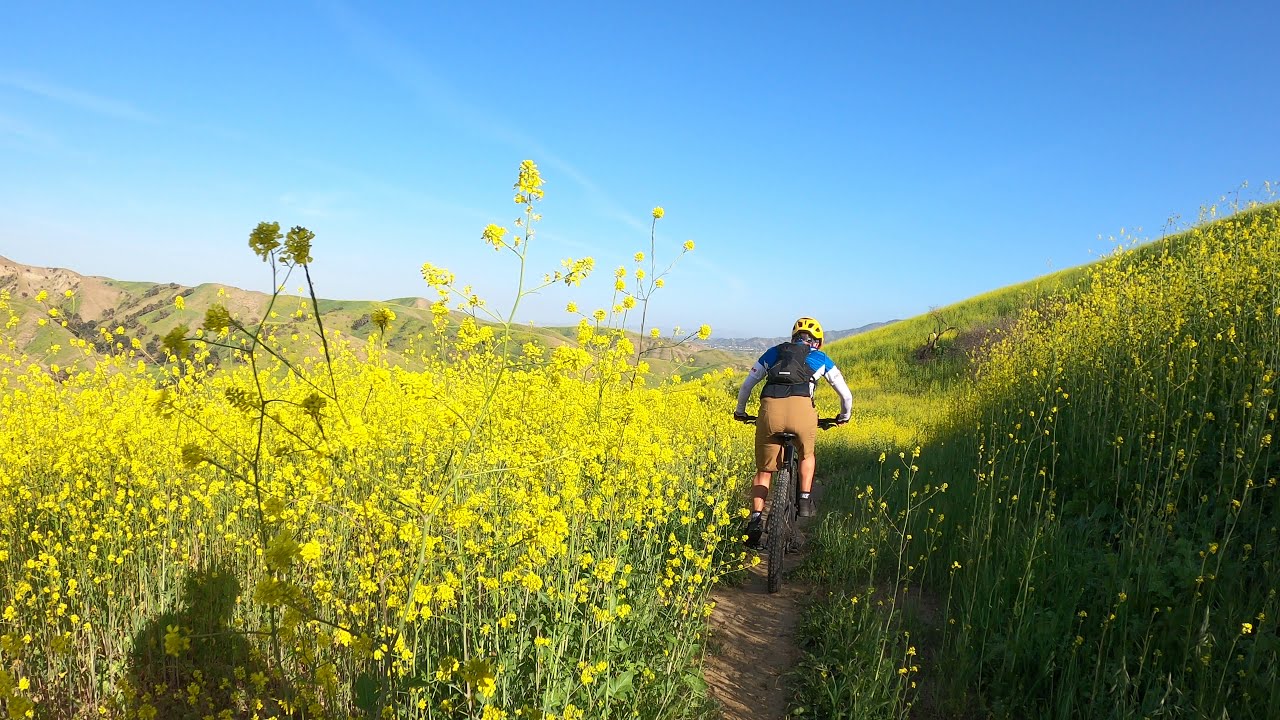The image captures a scenic outdoor moment on a clear, sunny day featuring a lone bicyclist navigating a narrow, well-trodden dirt path. The rider is wearing a yellow helmet, a blue shirt with white sleeves, brown shorts, black socks, black tennis shoes, and a black backpack. They appear to be riding a mountain bike, suggested by the thicker tires, through a field of tall yellow wildflowers, possibly resembling dill, that line both sides of the winding path. The flowers are vivid and plentiful, creating a striking contrast against the green grass and the occasional bare dirt patches on nearby hills. In the background, there are expansive hills and valleys, some covered in grass and trees, others barren. The sky is a breathtaking pale blue with minimal clouds, amplifying the beauty of the scene. A shadow on the lower left indicates the presence of another bicyclist, adding a subtle sense of shared adventure.